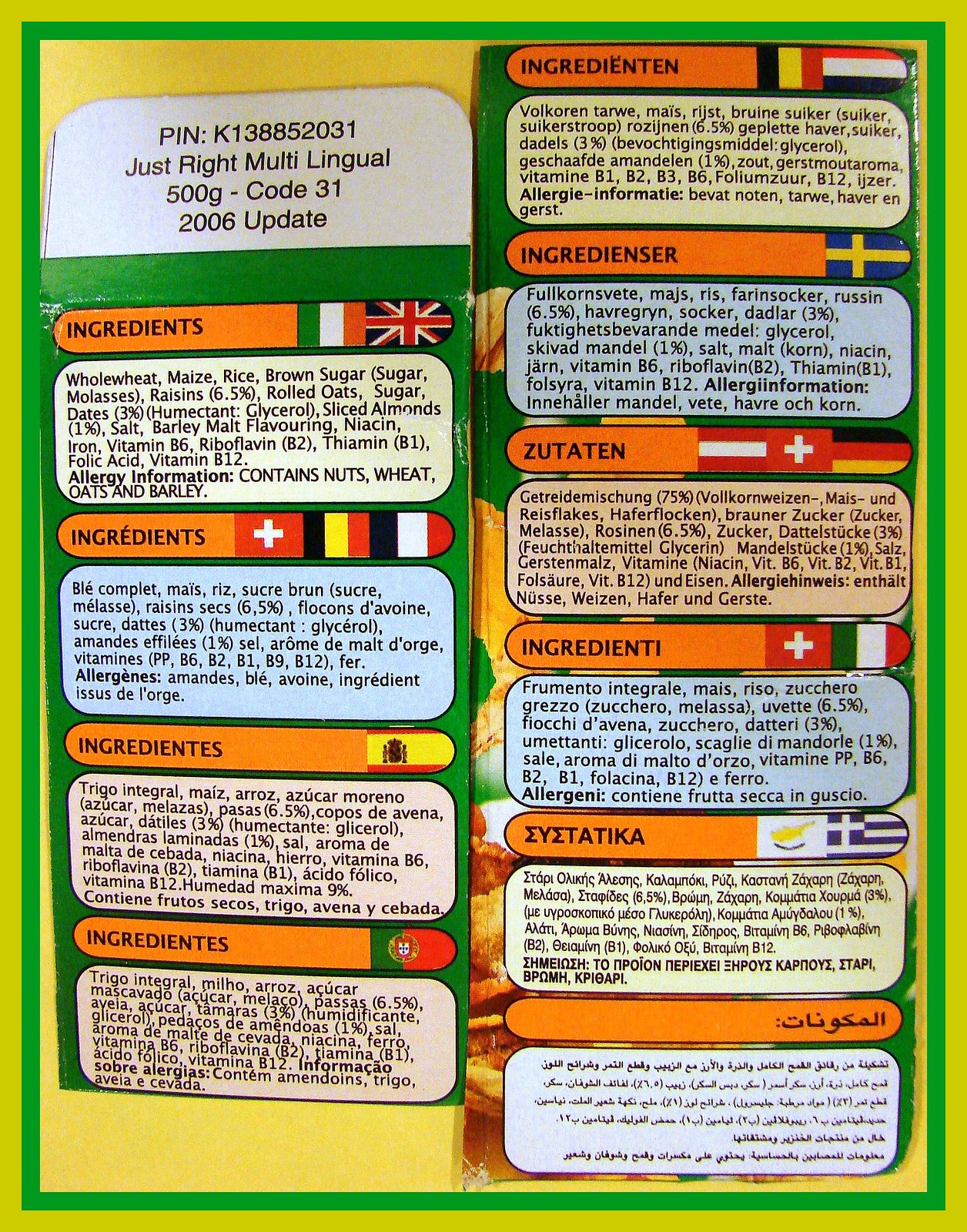The image portrays a detailed label from the back of a food packaging, prominently set against a yellow background with a green border. The main body of the label, which measures approximately 8 by 11 inches, features several blocks, each about 3 inches by 1.5 inches, bordered in green. Each block lists the word "Ingredients" accompanied by flags representing different nationalities. The first block lists ingredients in English, with the flags of the UK and Ireland. Subsequent blocks display the word "Ingredients" in multiple languages, each paired with corresponding national flags. The label showcases ingredients in ten different languages, emphasizing its multilingual aspect. In the upper left-hand corner, a white section displays a pin number along with details stating "multilingual, 500 grams, code 31, 2006 update." This information underscores the global accessibility of the product.